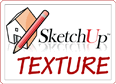This square-shaped close-up image captures an overhead view of a rocky road or walkway, where various sized rocks are embedded in a blackish-brown dirt mixture. The rocks, which are black, gray, slate-colored, and sometimes almost white or brown, create a textured and irregular pattern, giving it a collage-like appearance. Scattered throughout the image are pieces of dried, brown leaves and occasional twigs, adding to the natural debris. The rocks, in both jagged and smooth forms, blend seamlessly into the dirt, creating an overall composition of neutral earth tones dominated by dark blues and browns.